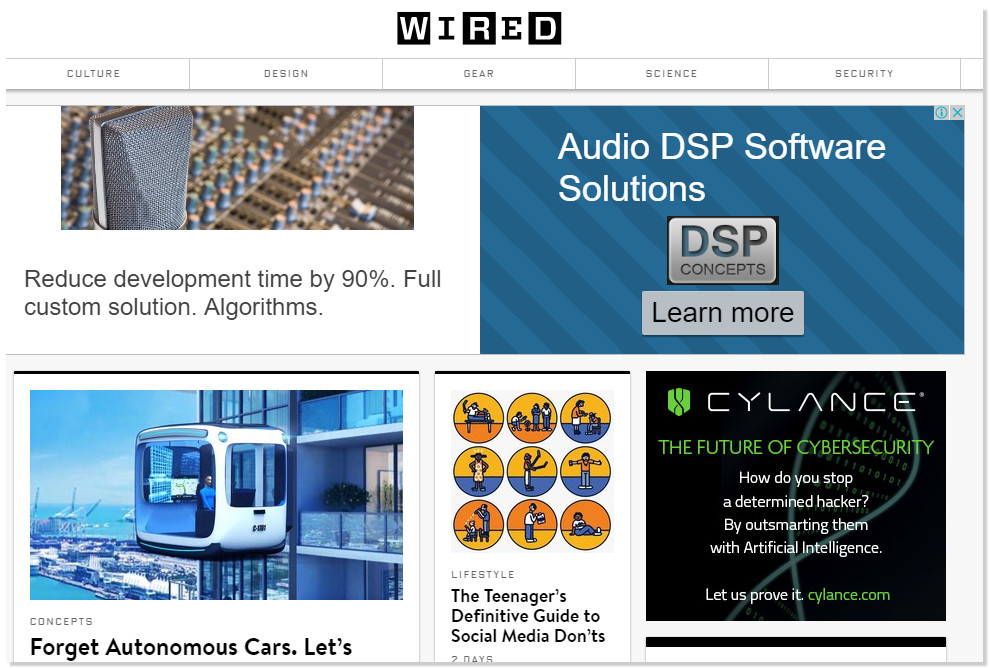This is a screenshot of the WIRED website, featuring a clean, white background. Centered at the top is the WIRED logo, which consists of the letters "W", "R", and "D" enclosed in black circles with white text, while the letters "I" and "E" are enclosed in white circles with black text. Directly below the logo is a navigation menu listing various sections of the website: "Culture," "Design," "Gear," "Science," and "Security."

Beneath this menu, there's a prominent photo depicting a computer processor. The accompanying text reads, "Reduce development time by 90%: Full custom solution algorithms." To the right of this image, a banner ad promotes audio DSP software solutions. The ad has a two-toned blue diagonal stripe background, with text in gray squares that states "DSP Concepts" and "Learn More."

Further down the page, there's an article section. The first article, labeled "Concepts," has a title that is cut off and reads, "Forget autonomous cars. Let's ..." This article is accompanied by an image of a seemingly futuristic outdoor elevator attached to the side of a building, though it is noted that the image was AI-generated. Adjacent to this is another article titled "The Teenager's Definitive Guide to Social Media Don'ts."